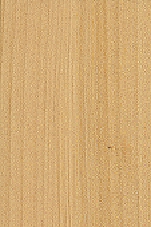This image is a close-up photograph of a light brown wooden board. The board features a smooth texture, likely treated, and displays a distinct wood grain pattern running vertically from top to bottom. The grain is fine, with closely spaced lines in the center and wider apart towards the left and right edges. Dark brown shading and several vertical streaks highlight the grain, adding depth and contrast. Notably, there are small, lighter-colored speckles throughout the wood, particularly noticeable in the top right section of the image. The overall appearance suggests a high-resolution, detailed depiction of the wood's natural texture and color variations.